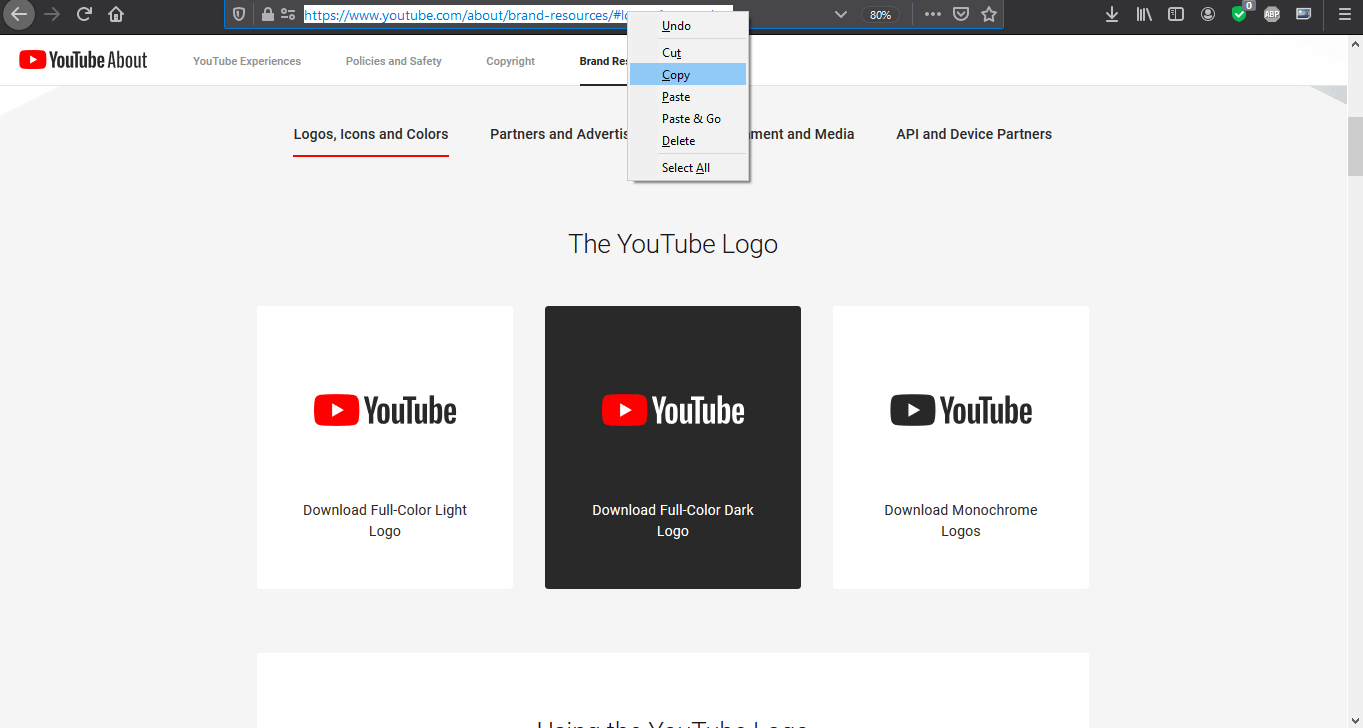A descriptive caption for the image:

The screenshot displays a YouTube webpage centered on brand resources. Starting from the top, a black banner features a left arrow, a right arrow, an undo button, and a home button. Below them is a white address bar with the URL "www.youtube.com/about/brandresources" in blue text. To the right of this bar, about 80% across, there is a star icon and a green box with a white check mark. Underneath, another white bar lists navigation links from left to right: "YouTube Experiences," "Policies and Safety," and "Copyright." In the top left corner, the YouTube logo is visible alongside the words "YouTube About." Below this, in bold black text, categories are listed: "Logos, Icons, and Colors," "Partners and Advertisers," and "API and Device Partners." Centered from the top, a dropdown menu shows options such as "Undo," "Cut," "Copy," "Paste," "Paste and Go," "Delete," and "Select All," with the "Copy" option highlighted in blue.